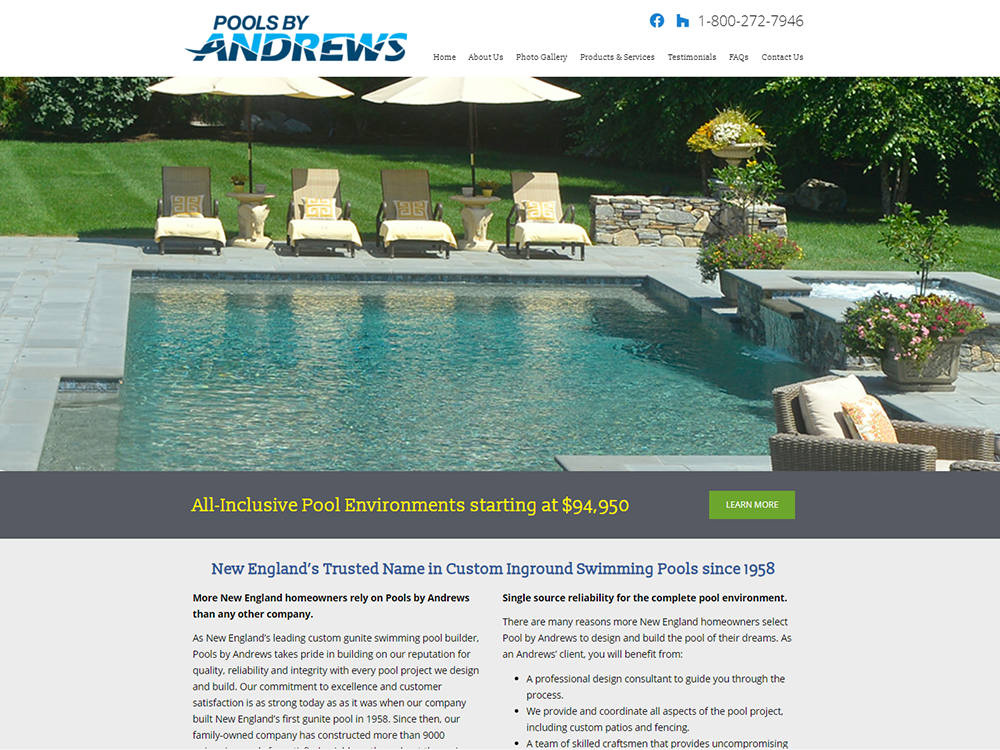**Detailed Website Caption: "Pools by Andrews"**

The screenshot showcases the home page of "Pools by Andrews." The company name is prominently displayed at the top in elegant blue text. Below, the image features a luxurious, square-shaped swimming pool. The pool is surrounded by a sleek stone deck area composed of gray stones. Stylish beige lounge chairs with matching pillows are strategically placed on the decking. Some of the lounge chairs are shaded by umbrellas, providing a touch of comfort and respite. 

To the right of the pool is an elevated jacuzzi, complementing the main swimming area. Enhancing the aesthetic are various planters filled with vibrant pink and red flowers. In the foreground, there is a cozy chair adorned with pillows, adding a homely touch to the scene.

The background presents a lush lawn bordered with an assortment of trees and decorative rocks, creating a serene atmosphere. Below the image, there is a highlighted green button that reads, "Learn More," directing potential customers to additional information. Just above this button, text indicates, "All-inclusive pool environments starting at $94,950."

Adjacent to the primary visual, a paragraph details the company's heritage, branding them as "New England's trusted name in custom in-ground swimming pools since 1958." It emphasizes that more homeowners in New England rely on "Pools by Andrews" than any other pool construction company. Additional text on the right explains the company's promise of "single source reliability for the complete pool environment," elaborating on their comprehensive approach to constructing custom pools.